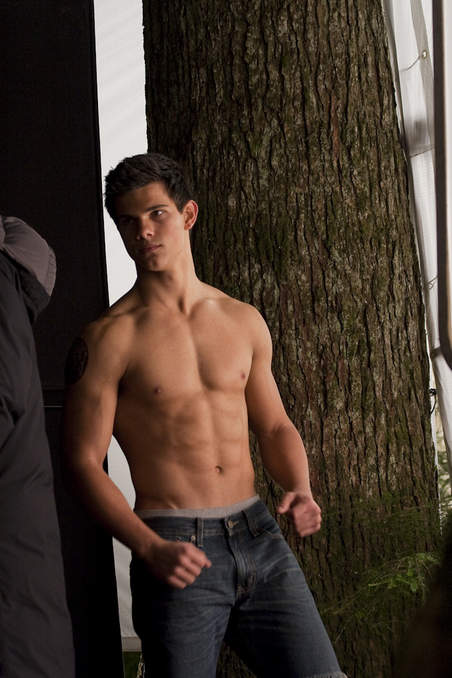This vertically aligned photograph likely portrays Taylor Lautner from his earlier 'Twilight' days, where he played the character Jacob. Lautner, appearing much younger, is posed shirtless with a strong, muscular build, and is dressed in blue jeans that reveal the edge of his light gray underwear. His hands are clenched into fists by his sides, giving him a ready-to-fight or intense posing stance. With serious expression, his brown eyes gaze to his right, and his short, dark hair is slightly spiked. He stands centered in front of a broad tree trunk, with another tree trunk visible to the left, creating a gap through which a light gray sky peeks through. The background includes small ferns at the base of the tree and additional elements like a sparse green bush. There are other indistinct items to the left side of the image, including what appears to be a black jacket and possibly some kind of panel or sail-like object. The image has a vertical crop, typical of a smartphone picture, adding to the candid and informal feel of the shot.